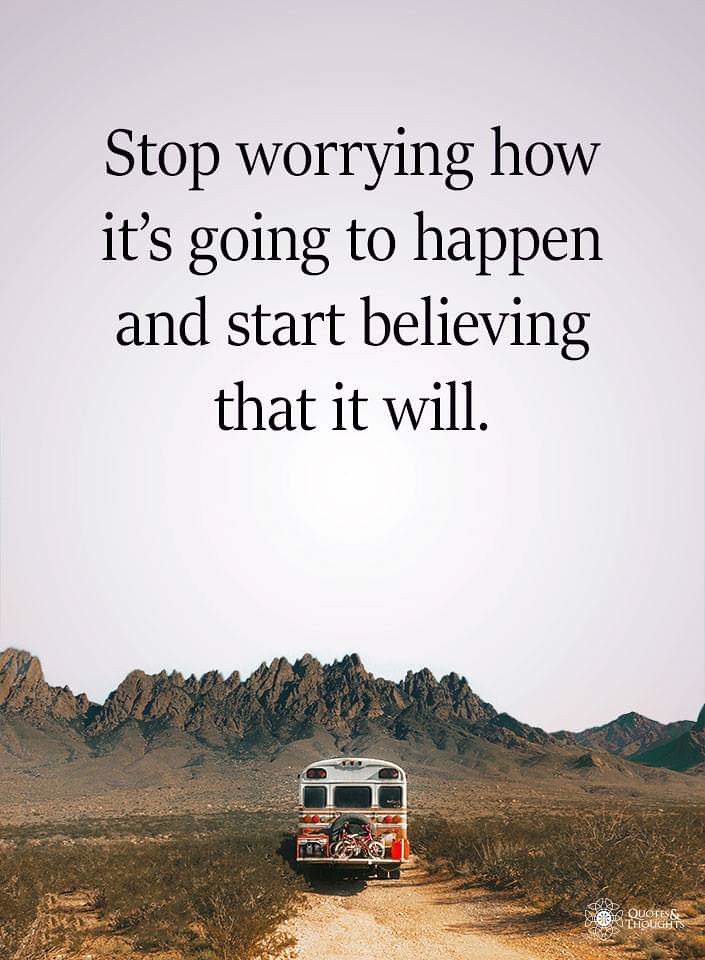This vertically rectangular poster showcases a serene and remote desert landscape. The backdrop features rugged, jagged mountains under a light purple sky, conveying an adventurous yet tranquil setting. At the bottom center of the image, a white, converted school bus, repurposed into a recreational vehicle, heads toward the mountains along a grassy dirt road. The back of the bus is fitted with a rack carrying bicycles and gas cans. The vivid scenery is emphasized by a palette of off-white, black, brown, red, orange, gray, and tan hues. Dominating the top of the poster is a motivational inscription in black print that reads, "Stop worrying how it's going to happen and start believing that it will," along with some smaller white text in the bottom right. This poster likely aims to inspire viewers to embrace the unpredictability of planning vacations and outdoor adventures.